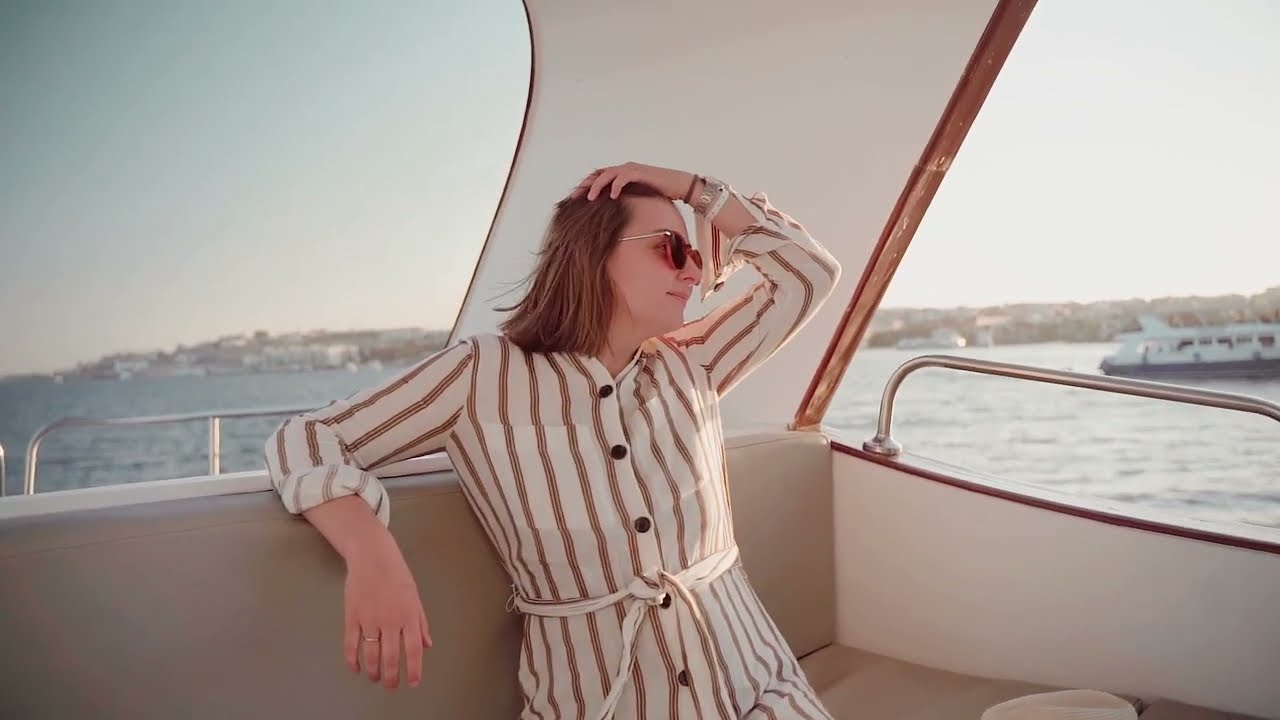In the photo, a woman with shoulder-length reddish-brown hair sits on a motor yacht. Her hair is parted slightly and she is running her left hand through it, pulling it back. She is dressed in a white and brown striped shirt with black buttons up the front and the sleeves rolled up. The woman has a light complexion and is wearing dark sunglasses, which shield her eyes from the bright sunlight. Her left arm, adorned with bracelets, rests on her head while her right arm is draped over the light brown cushioned seating of the mostly white boat.

She gazes off to her right, seemingly enjoying the serene atmosphere around her. In the background, other boats are anchored in the water, indicating that she is likely near a marina or harbor, with land and houses visible on low hills under a hazy sky. An old ferry is docked to the right side of the picture. The scene captures a peaceful and sunny summer day, perfect for a leisurely boat ride.